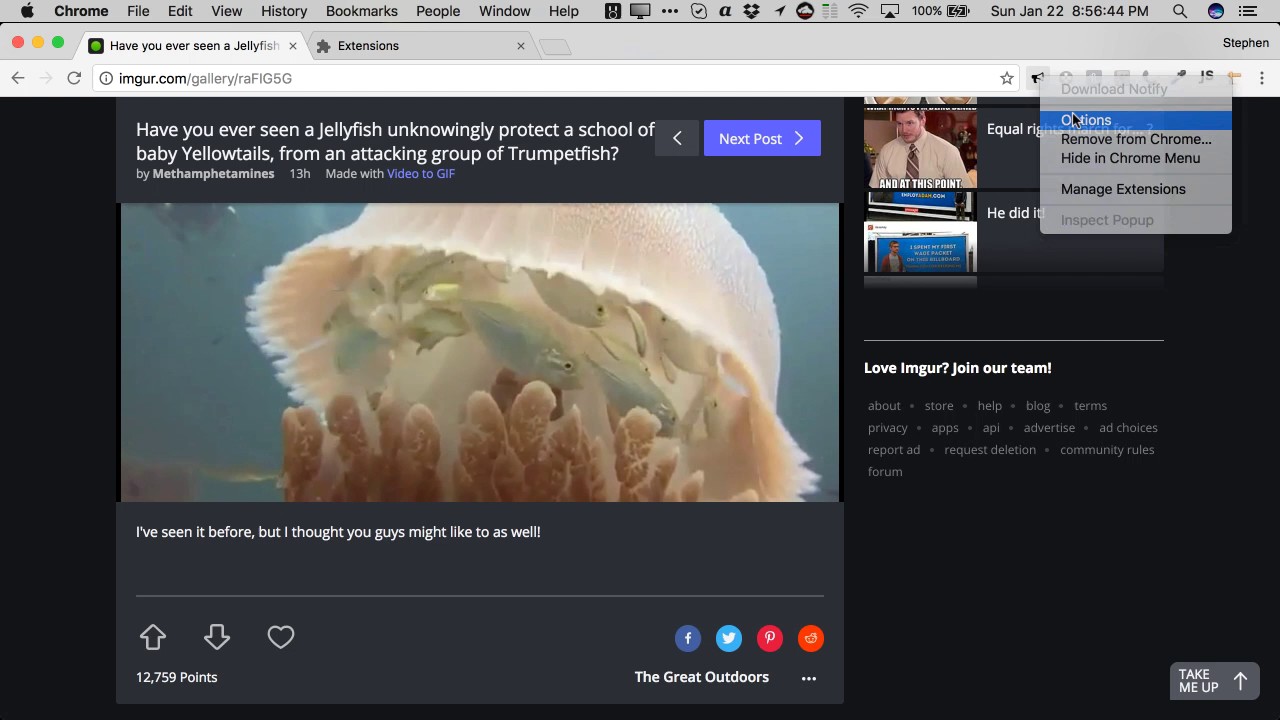Screenshot of a website displaying an imgur gallery.

At the top of the screen are two tabs: the first tab, selected and in a lighter gray, is partially labeled "have you ever seen a jellyfish...", while the second tab, not selected and in darker gray, has a gray puzzle piece icon and is labeled "extensions." Below the tabs lies the URL bar containing "imgur.com/gallery/raFIG5G".

The primary content of the webpage features a predominantly black background with a gray rectangular section at the center-left. At the top of this rectangle is white text reading, "Have you ever seen a jellyfish unknowingly protect a school of baby yellowtails from an attacking group of trumpetfish? By methamphetamines, 13 hours, made with video2gif", with "video2gif" highlighted in purple.

Centered within the gray rectangle is a photograph depicting a white jellyfish encircled by several small fish against a backdrop of pale blue water. Beneath the photo, white text states, "I’ve seen it before but I thought you guys might like to as well."

Further down, a thin gray dividing line separates the content. Below this line are interactive icons: a white upward arrow (upvote), a white downward arrow (downvote), a heart symbol, and the text "12,759 points." On the right side of these icons are social media sharing icons, and at the bottom-right of the gray box, it reads "The Great Outdoors" with a button featuring three dots next to it.